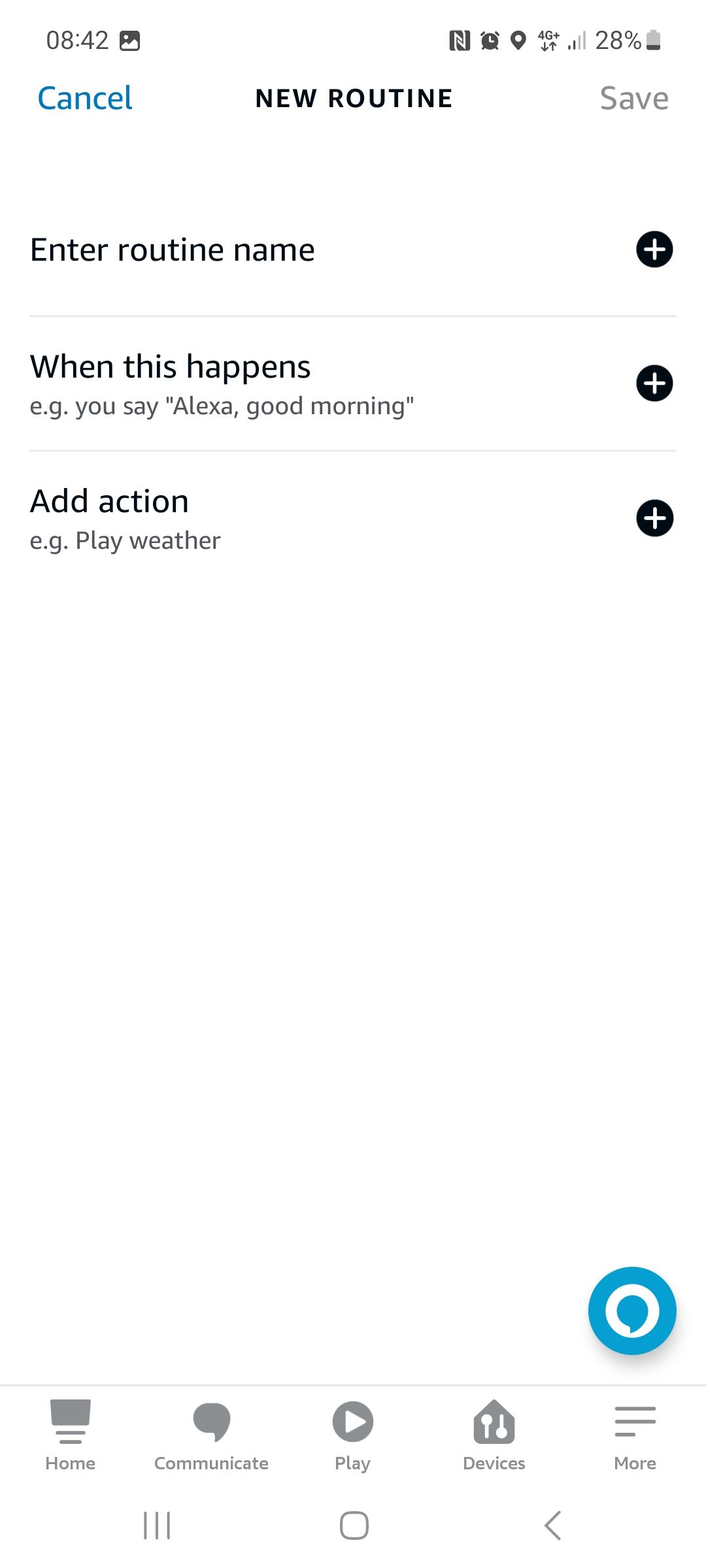The image captures a smartphone screen displaying a user interface for setting up a new routine in what appears to be an Alexa app. The screen is entitled "New Routine," with "New Routine" in bolded black capital letters. To the left of the title, in lowercase blue letters, is the word "cancel," and to the far right, in light gray lowercase letters, is the word "save."

On a clean white background, below the title, the interface includes a prompt with the text "Enter routine name," followed by a black circle featuring a white plus sign. Each section is separated by a light line.

Next, the section titled "When this happens" is below the routine name prompt. Underneath this, an example is provided: "e.g., you say 'Alexa, good morning'," followed by another black circle and plus sign.

Under the "When this happens" section, there's a section titled "Add action," with an example action of "Play weather." At the bottom right of the screen, the blue and white Alexa logo is visible. 

The lower navigation bar features options labeled "Home," "Communicate," "Play," and "Devices," arranged horizontally. The very bottom of the screen includes a small hamburger menu icon, a little square, and a gray arrow pointing to the left.